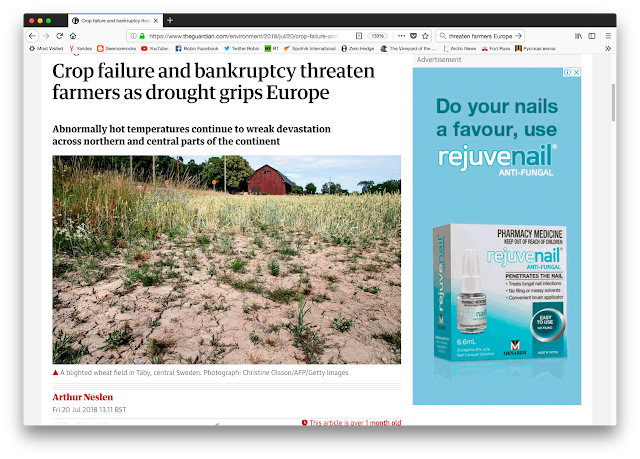A severe drought is gripping Europe's agricultural heartland, leaving vast expanses of farmland barren and desolate. Sparse patches of grass struggle to grow in the dry, cracked soil, emphasizing the harsh conditions that threaten the livelihoods of farmers facing the dual specters of crop failure and financial ruin. The image is framed by a black border at the top, providing a stark contrast to the parched landscape within the frame.